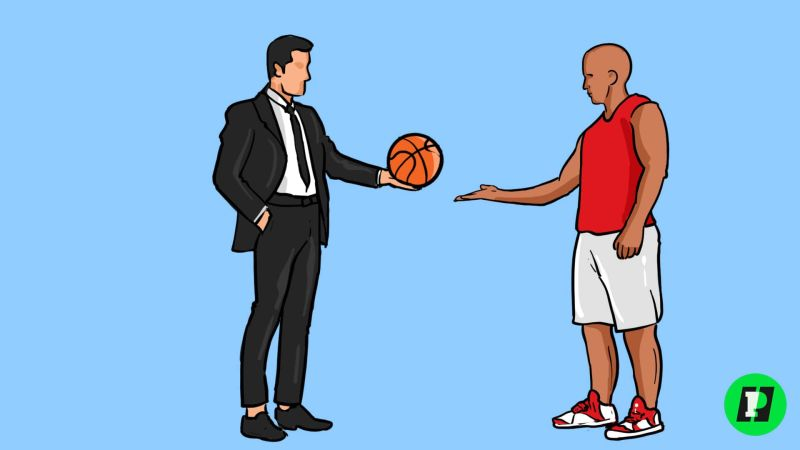This is a minimalist, stylized cartoon image set against a solid light blue background, depicting two figures interacting. On the left stands a white man in a black business suit, complete with a black tie and black shoes. He has short black hair and, notably, simple dot eyes. His hand is in his pocket while he hands a basketball to the other figure with his other hand. On the right, about the same height, is a dark-skinned man wearing red and white basketball shoes, white shorts, and a red sleeveless shirt. He has dot eyes but no hair. The scene is devoid of detailed context, enhancing its minimalist aesthetic, and a circular logo featuring a stylized pea and the letter 'P' appears in the bottom right corner. The composition suggests a transfer of the basketball, possibly symbolizing mentorship or a moment of transition.